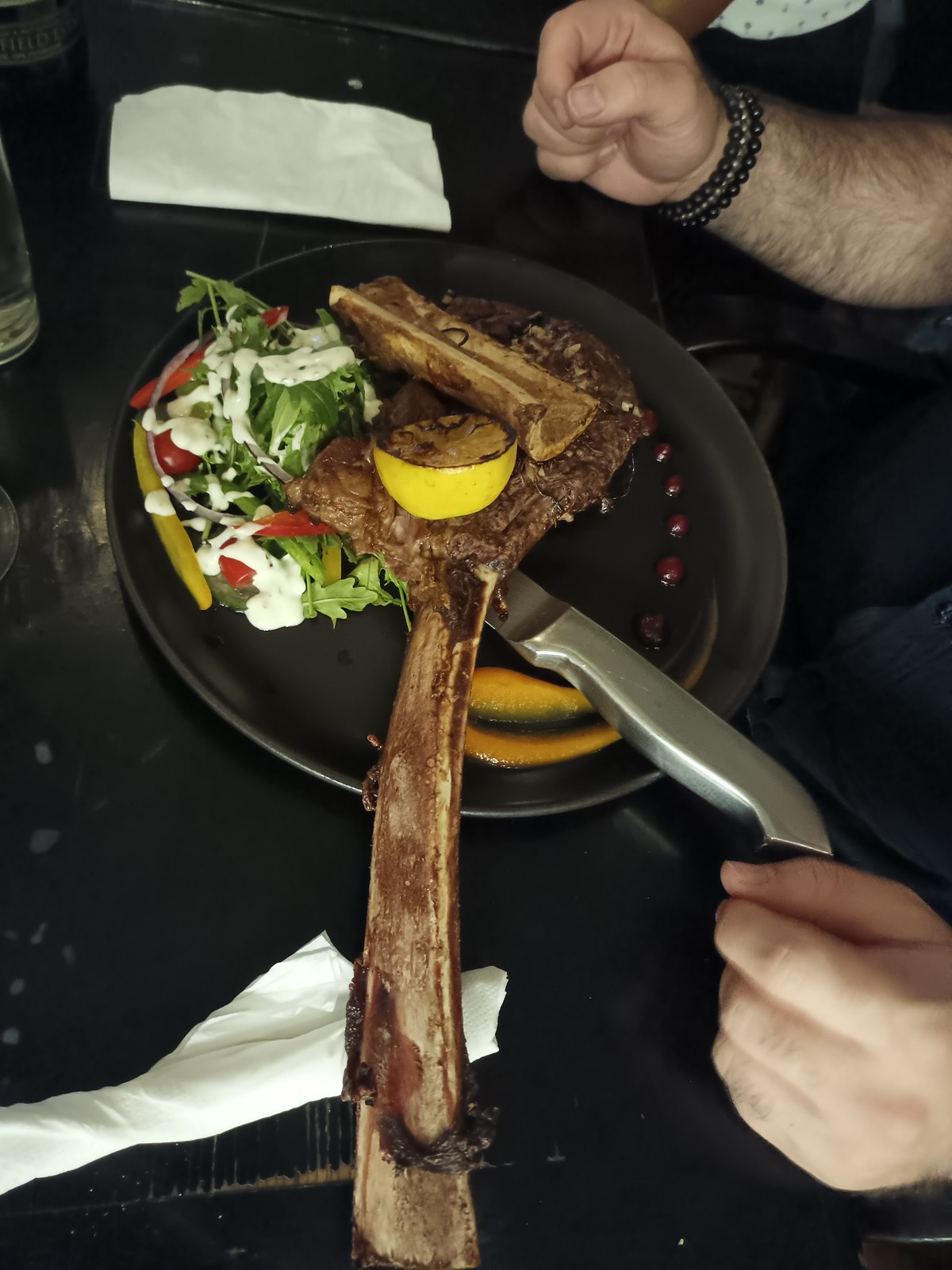A detailed image depicts a man, identified by his large, hairy forearms and hands, enjoying a meal at a black table. The focal point is a black plate that holds a substantial piece of meat with a long bone, possibly beef or lamb, accompanied by a seared lemon. Nestled beside the meat is a vibrant salad featuring green lettuce, red cherry tomatoes, orange carrot slices, and yellow banana pepper, all drizzled with creamy white ranch dressing. Next to the entrée rests a mysterious seared item, potentially a chunk of bamboo or mango. Surrounding the plate are several items: a silver knife positioned under the meat, a couple of white napkins, and what appears to be an additional frying pan nearby. The scene captures the essence of a hearty meal in progress, with a pair of hands and arms extending toward the food, their diverse textures indicating the presence of multiple people.